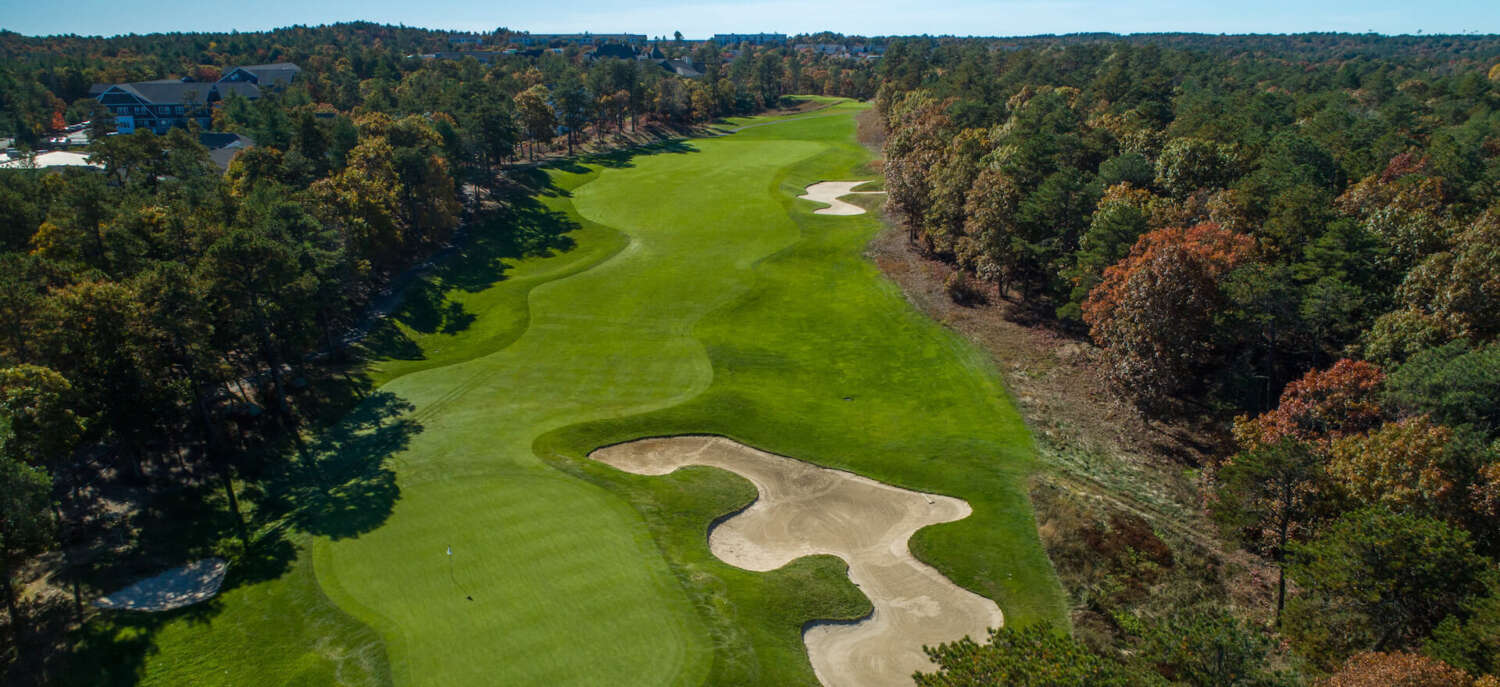This aerial photograph captures a long and narrow golf course that stretches into the distance, surrounded by dense forests that also extend far beyond the frame. The well-manicured grass of the course is characterized by slight hills and an irregular shape, with notable sand traps including a distinct one in the bottom middle that resembles the number three, and a smaller sand trap positioned above it. The lush greenery is interspersed with trees and bushes displaying hues of dark green and reddish colors, likely indicating autumn foliage. The left side of the image features a large building or possibly the clubhouse, with only its roof visible. The sky, a sliver of blue without clouds, forms the background for this very detailed and clear landscape image.